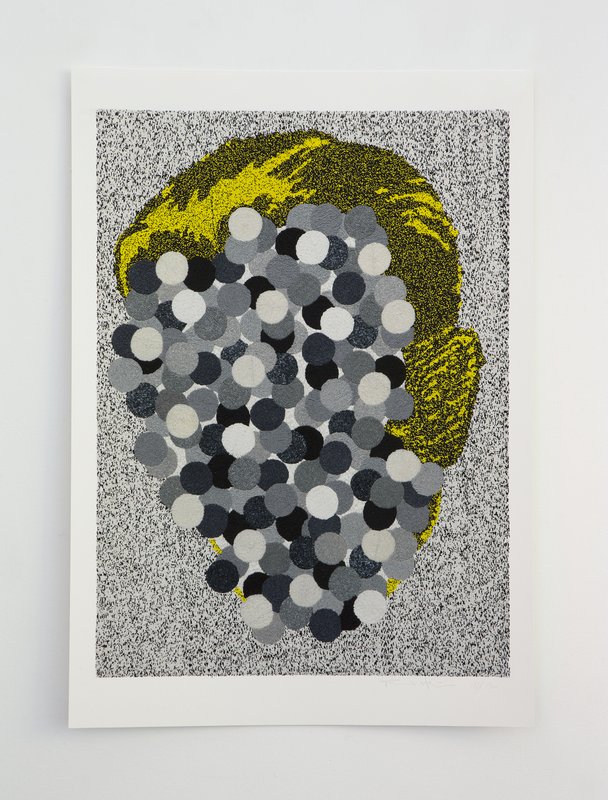The image is a vertically-oriented piece of artwork mounted on a white wall, surrounded by a white border, featuring a distinctive, abstract portrait. The background of the artwork appears as a pattern of black and white dots, reminiscent of TV static, which seamlessly merges into the depiction of a face. This face is oriented in profile, facing the left side of the image. The hair is illustrated in yellow and black to indicate shading, giving the impression of blonde hair, while the right side of the painting reveals a prominent ear with intricate black and gray lines. The face itself is abstractly covered in overlapping polka dots of varying shades from white to black, creating a layered, almost pixelated effect. These dots form irregular patterns over the entire facial area, giving it a textured appearance. The overall composition creates a striking, modern interpretation of a side-view portrait.